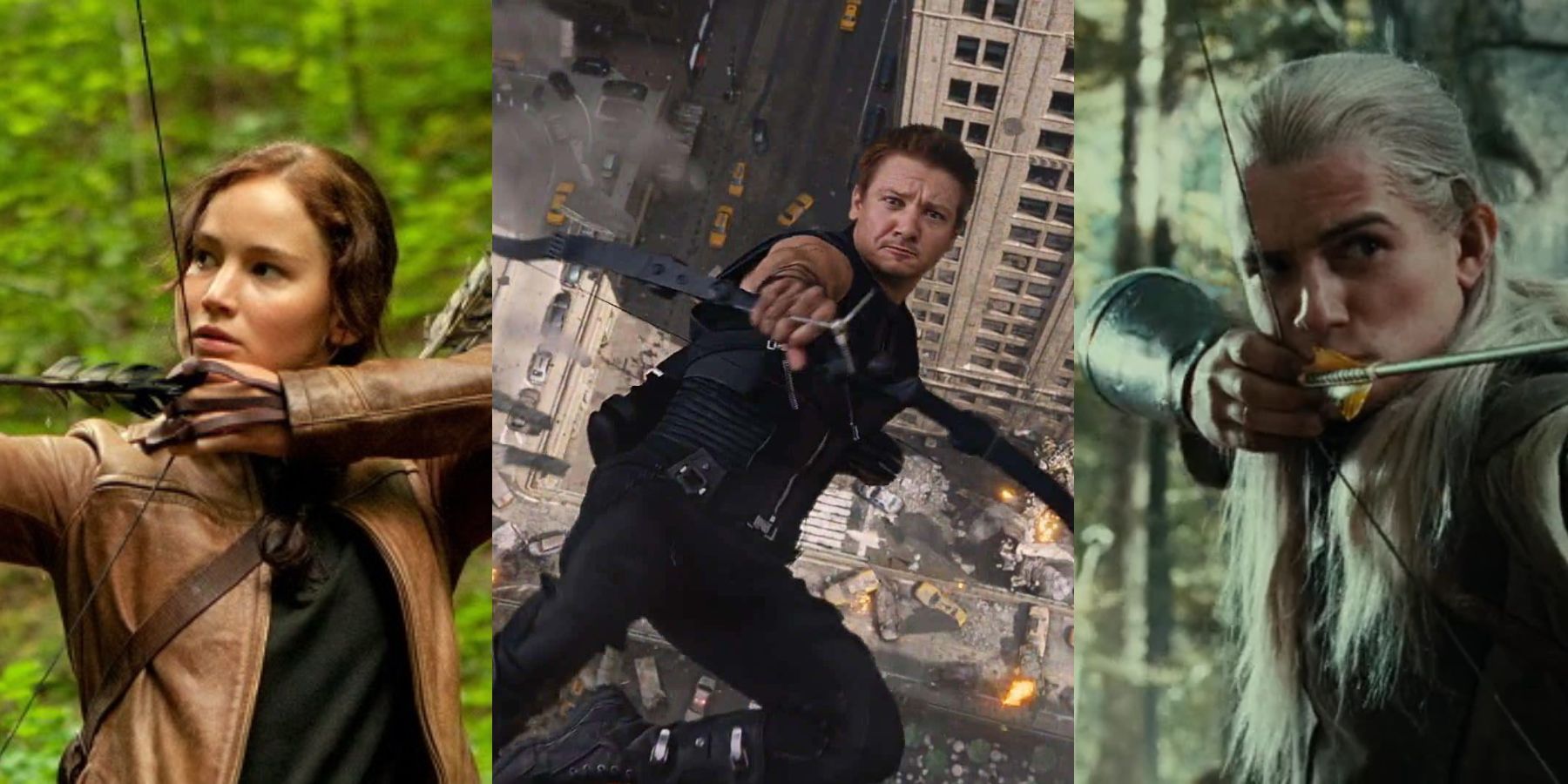This image is a rectangular, side-by-side arrangement of three archers from different movies, each holding a bow and arrow and looking serious. 

On the left, Katniss Everdeen from "The Hunger Games" stands facing left, ready to release an arrow. She is depicted in a vertical, portrait-oriented shot, donned in a brown leather jacket over a black shirt. The background is bright green, though slightly faded.

In the middle, the archer Hawkeye from "The Avengers" is captured in mid-freefall against a backdrop of a city street beset by destruction, with visible cabs and debris. Dressed in a black suit, he aims his bow upwards towards the camera.

On the right, Legolas from "The Lord of the Rings," with his long blonde hair, is also poised to shoot. Although his attire isn't visible in the frame, a leather arm guard and the orange fletchings of his arrow can be seen. The background behind him is faded, emphasizing his readiness.